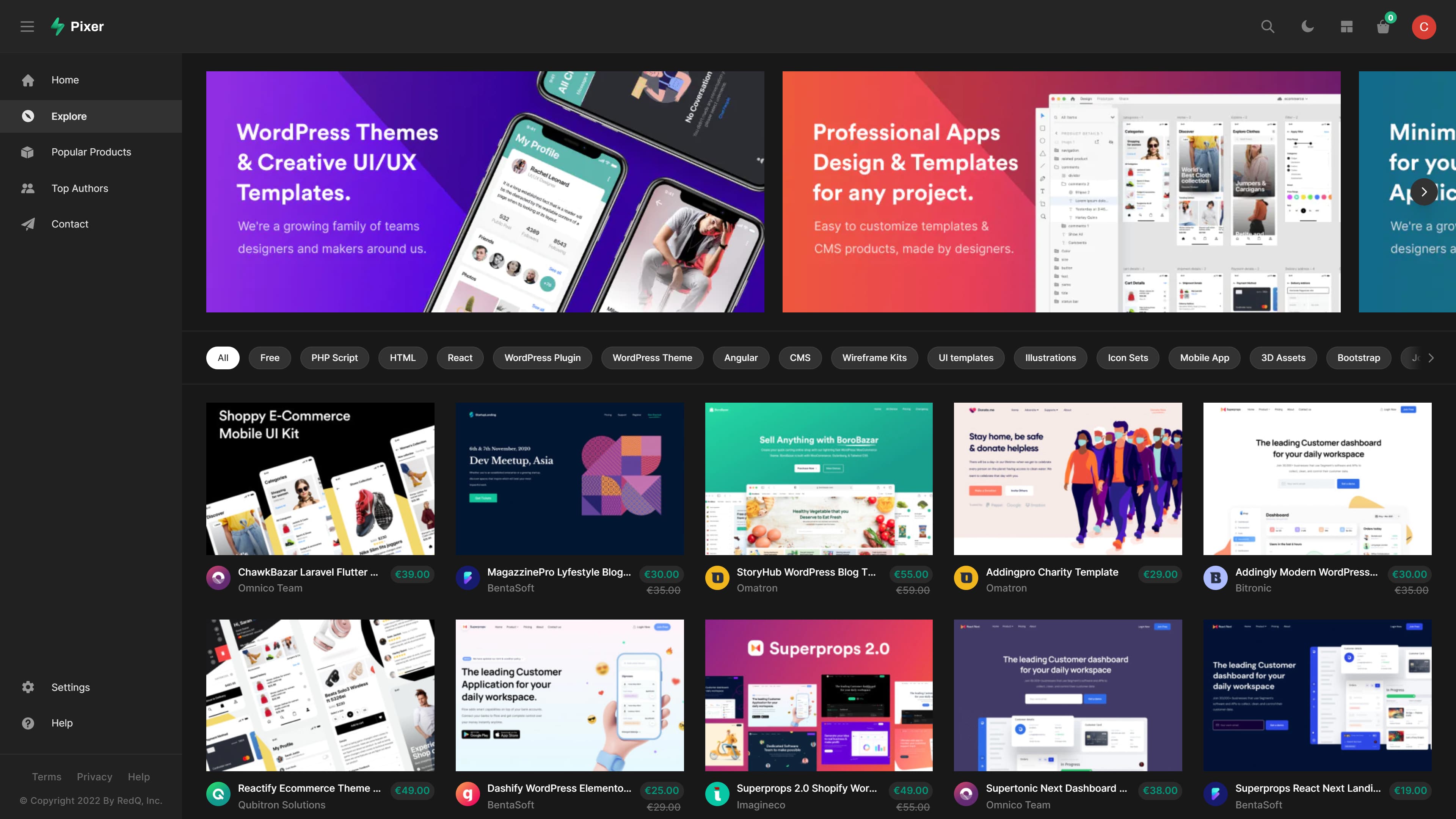The image depicts a black-themed WordPress website named "Pixer" as indicated by the logo positioned on the top left corner. Directly beneath the logo, a navigation menu lists several options: Home, Explore, Popular Products, Top Authors, and Contact. Centrally aligned at the top, there are two prominent banners. The first banner is labeled "WordPress Themes and Creative UI/UX Templates," while the second banner, located to its right, reads "Professional Apps Design and Templates for Any Project."

Below these banners, the website showcases a series of ten rectangular sections, each highlighting different product offerings. The first section advertises the "Shopee eCommerce Mobile UI Kit." Accompanying the title is the description "Chalk Bazaar Laravel Flutter" with a price tag of £39. Adjacent to this, the next section promotes the "Dev Meetup Asia" template by Magazine Pro Lifestyle Blog, priced at £30. The layout suggests that these are purchasable templates specifically designed for WordPress users.